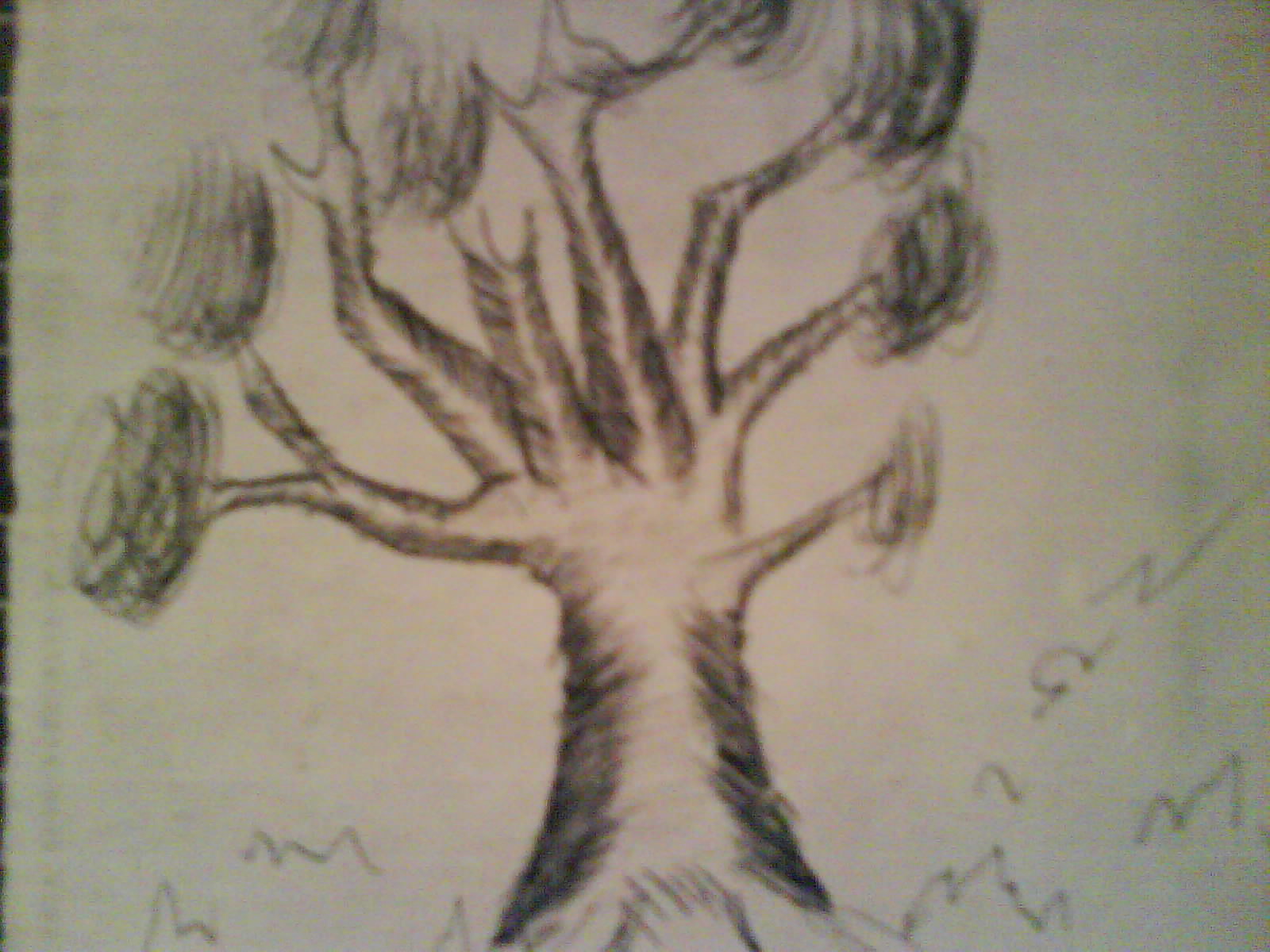This black-and-white drawing, likely created with a charcoal or pencil medium, features a cartoon-style tree on off-white or slightly gray paper, influenced by surrounding lighting. The tree's thick, shaded trunk extends upward, lightening in its center, and branches out into seven or eight primary branches. Each branch splits further, at varying angles, into secondary branches with swirled, circular, and oval shapes representing foliage at their ends. The branches, especially one at the top, evoke whimsical characteristics reminiscent of Dr. Seuss illustrations. The background has minor, unreadable symbols along the bottom and right side, adding to the drawing's unique texture and depth. The entire composition is subtly lit by a reddish hue, casting a gentle reflection on the paper.